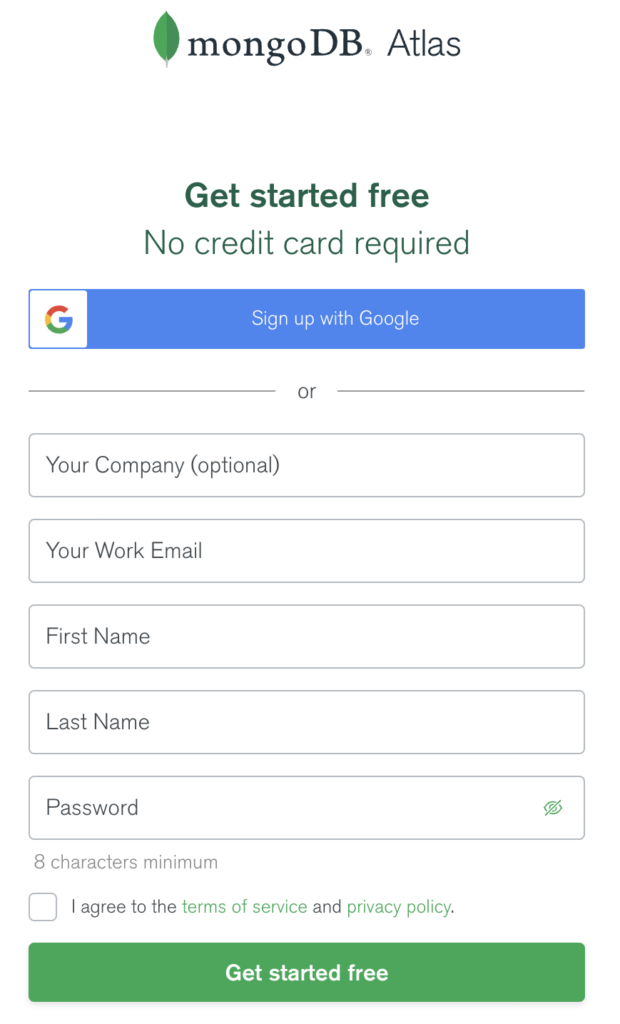The image displays the 'Create Your Account' screen from the MongoDB Atlas website. At the top center, the header reads "MongoDB Atlas" with a small, green leaf icon to its left. Just below, the text "Get started free, no credit card required" is prominently displayed. Consecutively, there’s a blue button featuring the Google "G" logo on its left side with the white text "Sign up with Google" inside the button. 

Underneath this option, the word "or" is centered, which leads into several text fields organized vertically. These fields are labeled respectively as: 
1. "Your Company" (with "optional" in parentheses)
2. "Your Work Email"
3. "First Name"
4. "Last Name"
5. "Password" (accompanied by a small eye icon on the right side for viewing the entered password)

Below these fields, outside the boxed area, the text "Eight characters minimum" is indicated. Further down on the left side is an unchecked box next to the statement "I agree to the terms of service and privacy policy," reinforcing the need for user agreement. Finally, at the bottom of the form, a green "Get Started Free" button invites users to proceed.